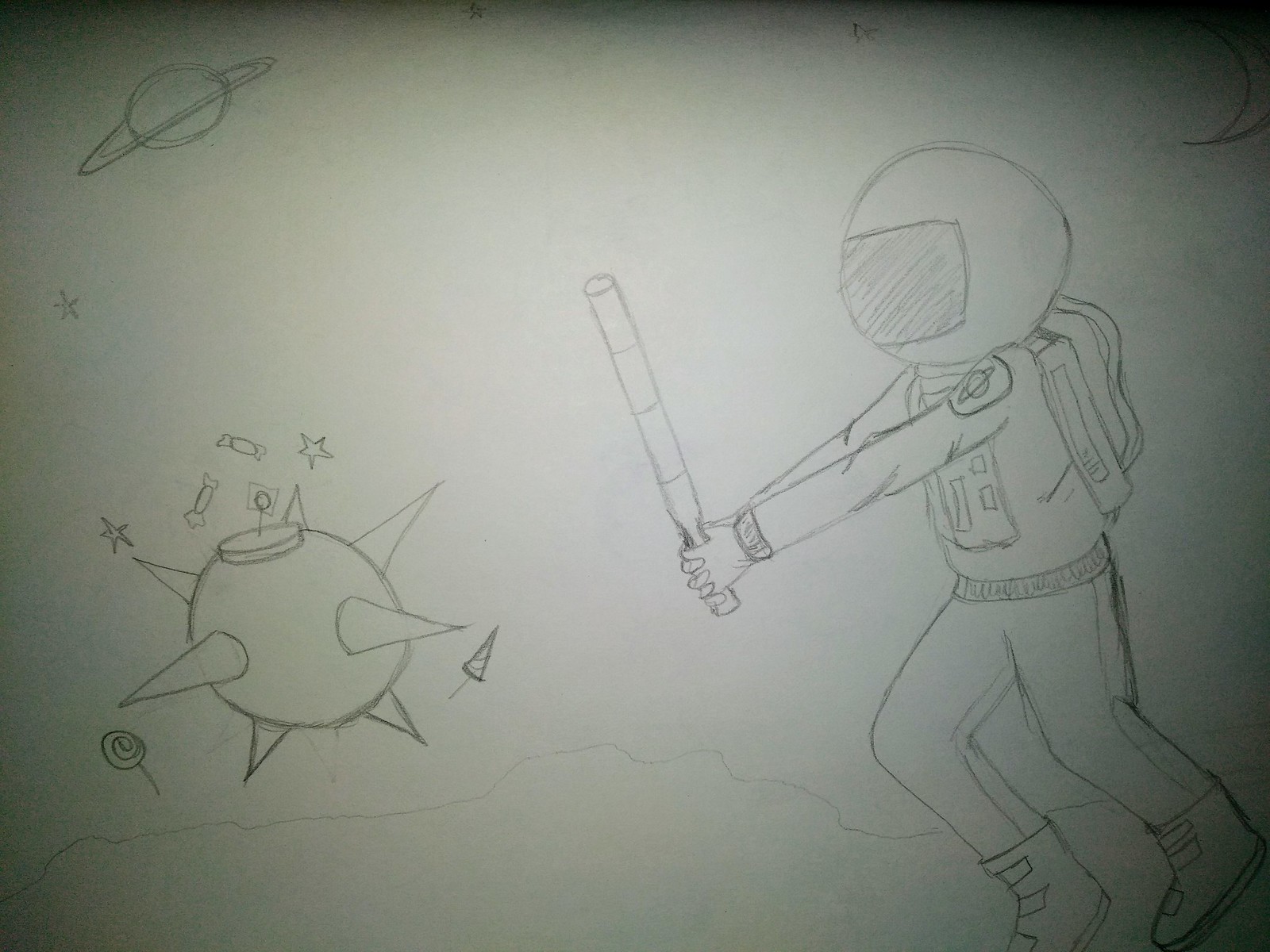This charming hand-drawn sketch presents a whimsical and imaginative scene set against the backdrop of outer space. At the heart of the illustration is an astronaut, striking a dynamic pose as they swing a baseball bat. Contrary to typical portrayals of space exploration, this astronaut engages in an unexpected activity, adding a playful twist to the scene. The spacesuit worn by the astronaut is intricately detailed, featuring an array of elements such as mission patches, an external backpack, and interconnected tubes, all contributing to a sense of realism. The helmet is large and rounded, equipped with a shaded visor that obscures the astronaut's face, enhancing the mystery.

In the background, the artist has skillfully included a variety of celestial bodies that add to the whimsical nature of the image. A cartoonish sun beams with exaggerated rays, while other space debris like a spiky ball floats nearby, creating an engaging and fantastical universe. This delightful juxtaposition of the mundane with the extraordinary captures the viewer's imagination and brings the scene to life.